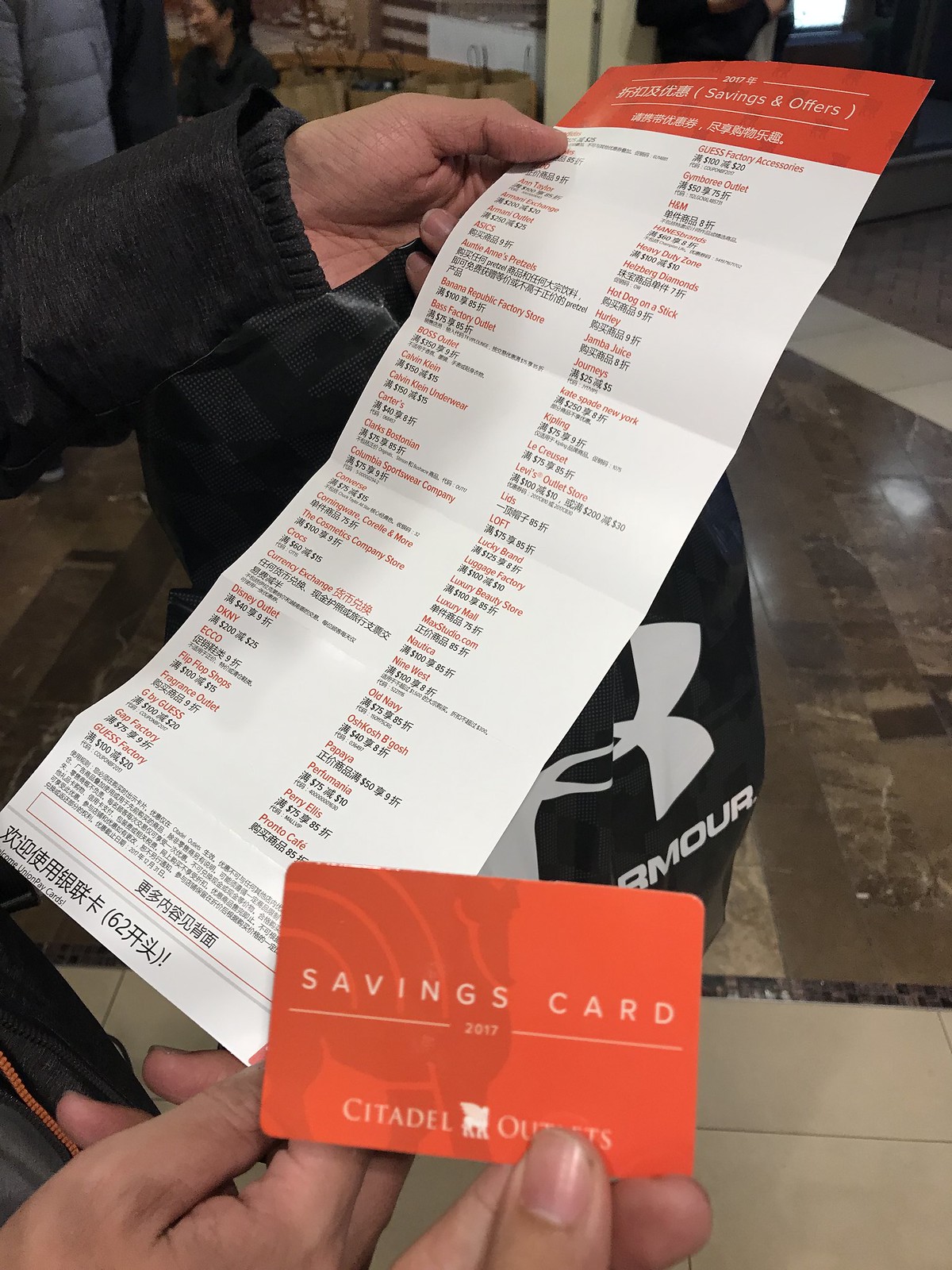The image depicts a person holding a menu, written in what appears to be Chinese characters. The menu itself features a white background and a red header at the top. The individual's left and right hands are visible, with the right hand emerging from the bottom left side of the frame holding the lower part of the menu, and the left hand extending from the top left side grasping the upper part. Additionally, a third hand is seen coming from the middle lower portion of the image, holding what seems to be a savings card.